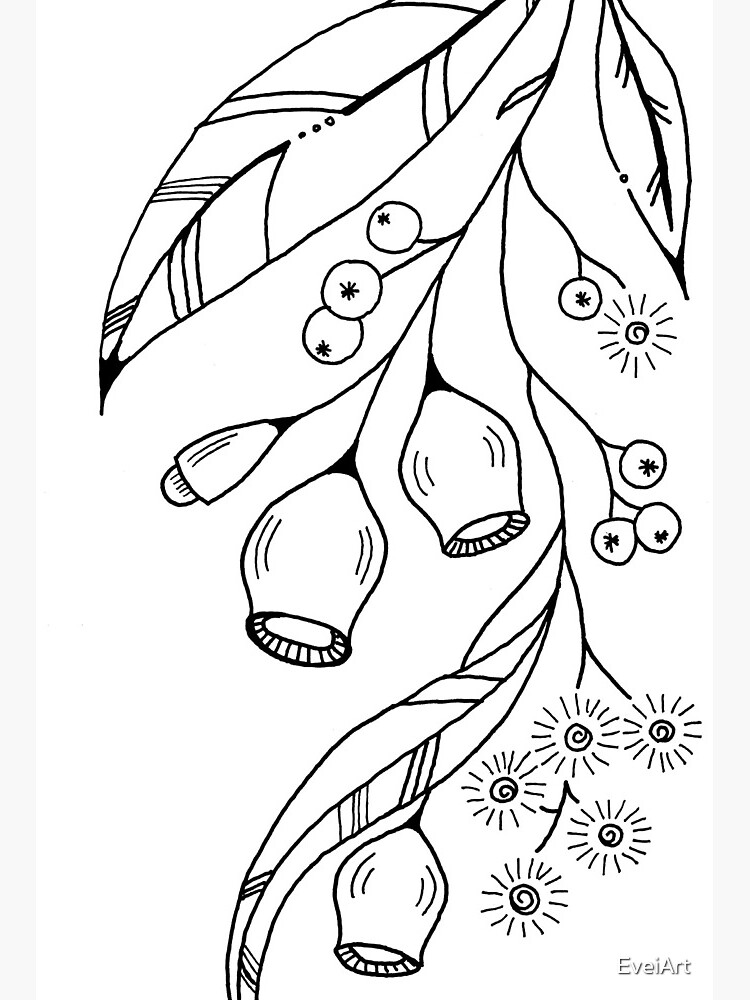This artist's rendition of a vine, titled "Evvy Art" in the lower right-hand corner, is a black and white line drawing set against a white background. The composition is vertical, with the vine depicted hanging upside down from a branch that extends from the top of the image. The vine features narrow, long leaves that cascade downward, interspersed with round berries and flowers. The flowers, which resemble the tops of wine glasses, are intricately outlined and contribute to the delicate aesthetic. The artist's detailed black lines contrast sharply with the white background, emphasizing the variety of natural elements, including leaves, berries, and flowers. The lack of color in the monochrome palette highlights the intricate design and offers potential for coloring or tracing.